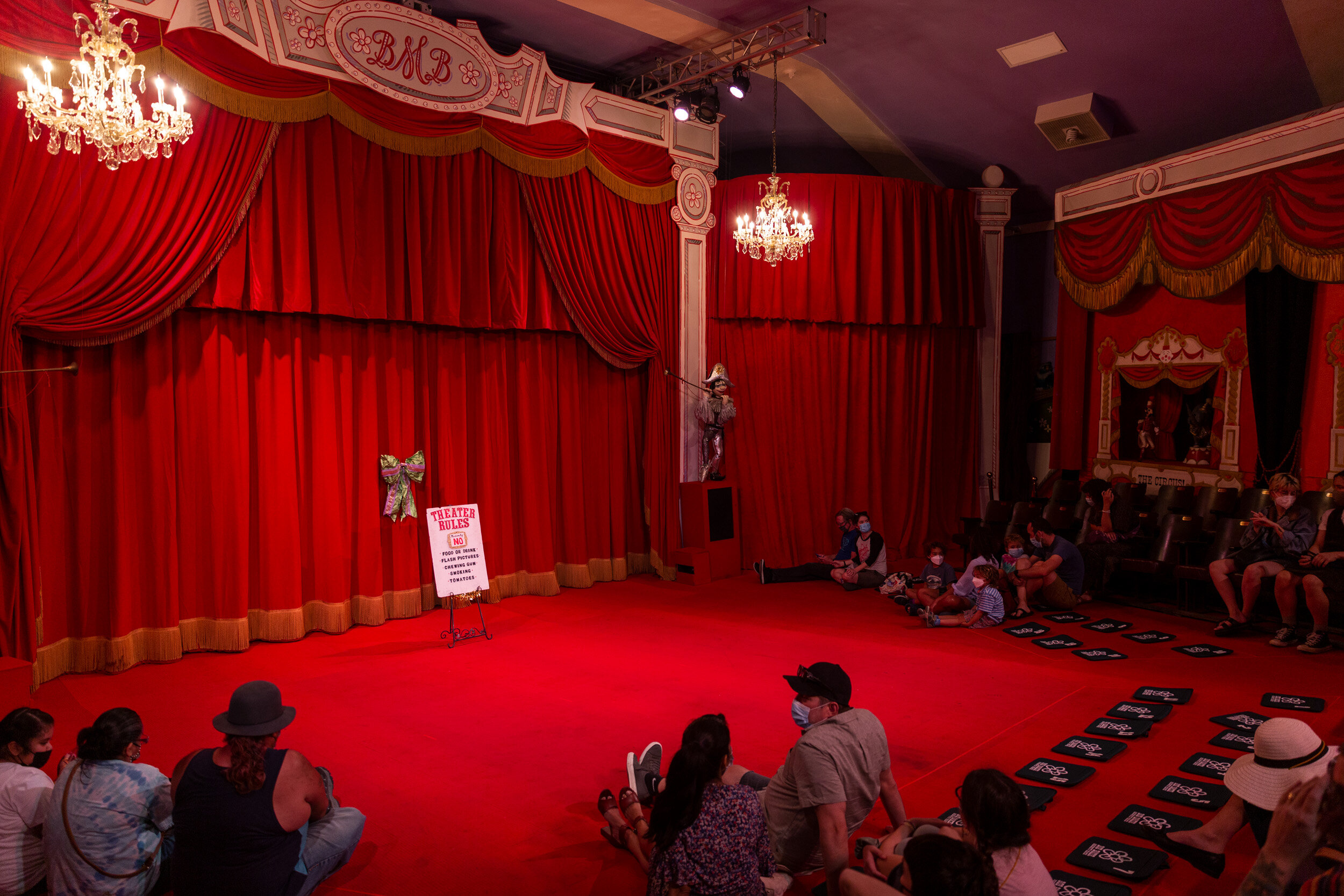The image depicts the interior of an ornate theater, lavishly decorated in striking shades of red and gold. The stage, draped in crimson velvet curtains adorned with gold and purple bows, is identified at the top with a flowery, western-designed BMB logo. Two grand golden chandeliers hang elegantly on either side of the stage, casting a warm glow over the space.

The center stage features a prominent sign listing the theater rules: "No food or drink, no flash photography, no chewing gum, no drinking, and no tomatoes." Below the sign, the floor is covered in a rich red carpet where people are seated cross-legged, most of them masked for COVID-19. These patrons include families, with children and women wearing hats, all seated comfortably on small pads instead of traditional chairs.

The overall ambiance is one of opulence and grandeur, with every detail contributing to a very ornate and fancy atmosphere. The curtains remain closed, suggesting that the performance has yet to begin. The detailed interior includes a small statue atop a red table, enhancing the theater's sophisticated decor.